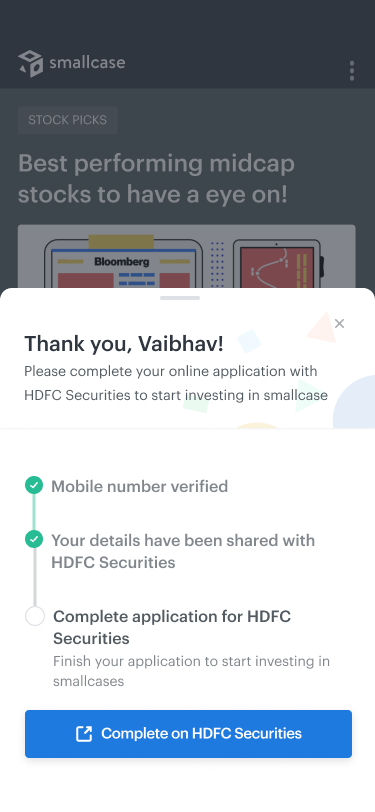This image is a detailed screenshot from a phone application called "Smallcase." At the top of the screen, there is a black text box with the word "Smallcase" accompanied by a small box icon. Towards the right side of this header, three vertical dots indicate more options.

Just below this header, there is a dark gray box labeled "Stock Picks," which is followed by a subtitle reading "Best performing mid cap stocks to have an eye on." The top portion of a white box beneath this section displays stock graphs and includes the label "Bloomberg."

The majority of the screen is occupied by a white message box, constituting about two-thirds of the display. This message, addressed to an individual named Vaibhav, says, "Thank you Vaibhav!" with both a question mark and exclamation point, indicating a friendly yet urgent tone. An 'X' button on the left side allows the user to close the message box. 

The message instructs the user to complete their online application with HDFC Securities to start investing in Smallcase. Below this directive, there is a thin line separating the instructions from three checklist items accompanied by little circles.

1. The first item, "Mobile number verified," has a green checkmark indicating its completion.
2. The second item, "Your details have been shared with HDFC Securities," is also marked with a green checkmark.
3. The final item, "Complete application for HDFC Securities," is not checked off and urges the user to "Finish your application to start investing in Smallcase."

At the very bottom of the screen, there is a prominent blue button labeled "Complete on HDFC Securities," with a small box to the left containing an arrow pointing to the right, suggesting a forward navigation link.